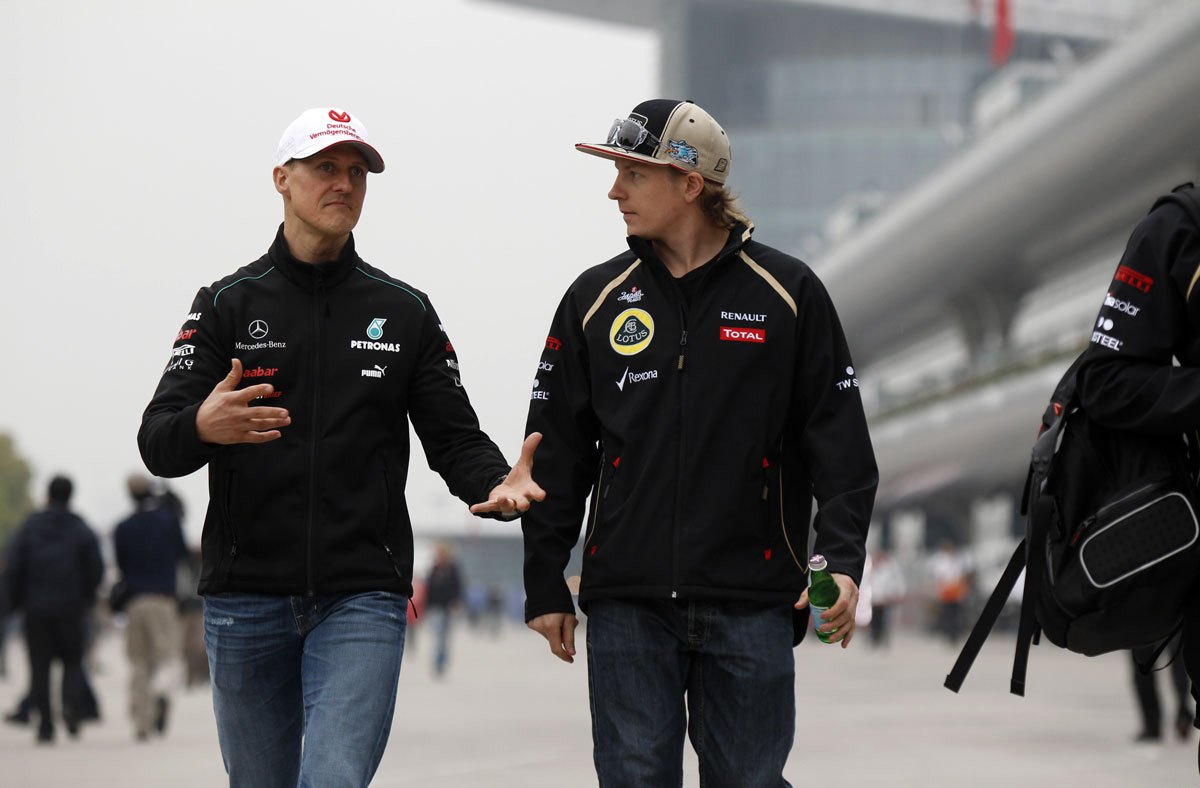In the photo, two men are walking towards the camera, appearing to be deeply engaged in conversation. Both are wearing baseball caps and black jackets adorned with several sponsor logos, including Mercedes-Benz, Puma, and Protomas, indicating they might be professional race car drivers or part of a racing team. 

The man on the left, slightly older, wears a white baseball cap and blue Levi's jeans. He has his hands out as if explaining something to his companion. The man on the right, younger by about 10-15 years, dons a white and black baseball cap with sunglasses resting on the bill. His jacket is distinguished by yellow lines on the shoulders, and he carries a green Pellegrino bottle in his left hand. Among the crowd in the background, partially visible, is another individual dressed in a similar racing outfit, carrying a backpack. The setting suggests a vibrant, possibly bustling, environment associated with a racetrack event.